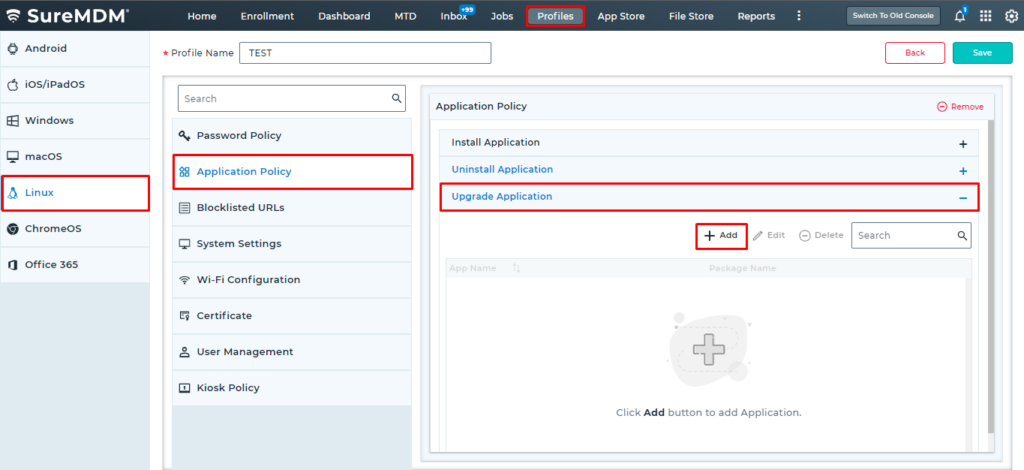The image depicts a detailed screenshot of the SureMDM web interface. In the top left corner of the interface, there's a thin, dark banner, transitioning from black to pale dark blue, featuring white text that reads "SureMDM.” Below this banner, the webpage is predominantly white with sections that display navigation options, including "Home," "Enrollment," "Dashboard," "MTD," "Inbox," "Jobs," "Profiles," "App Store," "File Store," and "Reports." 

To the far right, there are additional interface elements: an options button, a grid icon with four squares, a notification bell with a blue circle containing the number "1," and a light gray button labeled "Switch to Old Console" with white text.

Above the "Inbox" section, a blue rectangle with white text displays “+99.” The primary background of the website features a mix of white and light blue colors. On the left side, a column lists various device categories: "Android," "iOS," "iPad OS," "Windows," "Mac OS," "Linux," "Chrome OS," and "Office 365." Adjacent to this column, another column includes a search bar at the top followed by options like "Password Policy," "Application Policy," "Blacklist URLs," "System Settings," "Wi-Fi Configuration Certificate," "User Management," and "Kiosk Policy."

The right-hand main section of the image focuses on the "Application Policy" area, where a rectangular section contains smaller buttons for "Install Application," "Uninstall Application," and "Upgrade Application." A red rectangle highlights several elements: the "Profiles" option near the top of the page, the "Linux" section in the left column, "Application Policy" in the adjacent column, and specifically the "Upgrade Application" in the central area. Below this, an "Add" button is prominently highlighted in red.